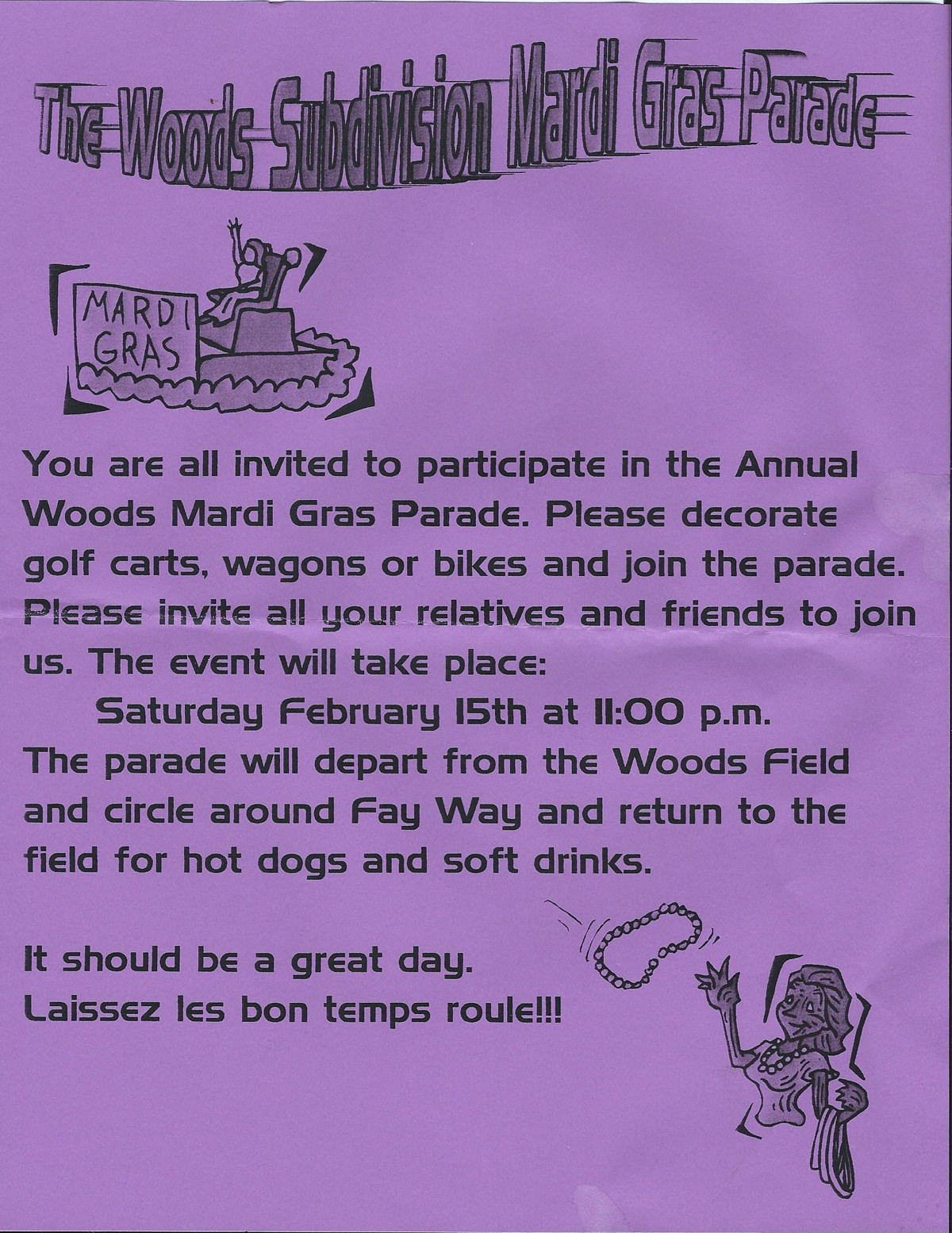The invitation is printed on purple paper with black text and a lighter gray title at the top that reads, "The Woods Subdivision Mardi Gras Parade." Beneath the title is a cartoon image of a lady on a float with the word "Mardi Gras" prominently displayed. The text invites everyone to participate in the annual Woods Mardi Gras Parade, encouraging the decoration of golf carts, wagons, or bikes. Attendees are asked to invite their relatives and friends. The event is scheduled for Saturday, February 15th at 11 p.m. The parade will start from Woods Field, circle around Faye Way, and return to the field where hot dogs and soft drinks will be provided. The phrase "Laissez les bons temps rouler," a French saying that means "Let the good times roll," is included in the invitation. In the bottom right corner, there's another animated image of a woman tossing a necklace of beads into the air with her right arm, while more necklaces are draped over her left arm.